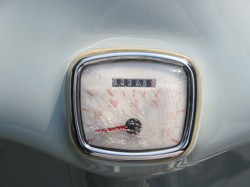The image depicts a small, somewhat grainy photograph of what appears to be a vintage speedometer, likely from an old car. The speedometer is housed in a metal frame, suggesting it was once part of a classic vehicle. The metal has an aged, faint light blue hue, almost white but just tinged with the slightest blue. Surrounding the face of the speedometer is a cream-colored ring encased in a stainless steel silver frame, reminiscent of the shape of old tube TVs.

The speedometer's dial has a white background, akin to a clock face, accented with red speed markings. The mileage counter is an old-school mechanical type with rolling wheels that display numbers. The counter shows a sequence where the first five digits are in black and the last digit is in red, reading "033469." 

Additionally, the speedometer features a traditional gauge with a black circle and a red pointer needle indicating speed, though the readability is compromised by the cracked and crackled glass covering it. This aged and weathered appearance adds to the overall vintage aesthetic of the piece.